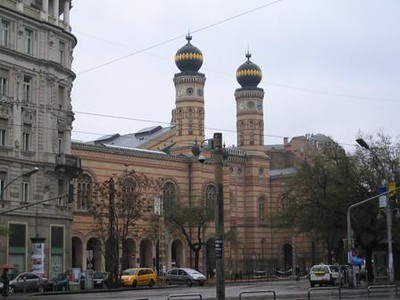In the image, a large, multi-story building sits prominently in the center, painted in light orange and tan hues. The structure is crowned by two minarets featuring black and golden onion domes with pointy tops. A tall metal pole with lights stands centrally within the frame. To the left of the main building, there's a grey, equally aged building. The foreground shows a bustling street filled with cars, including a noticeable yellow one near the bottom center. Both the left and right sides of the image are dotted with trees. Additionally, power lines crisscross the scene, and street lamps are scattered around. The sky above is bright and almost white, contributing to the well-lit atmosphere.